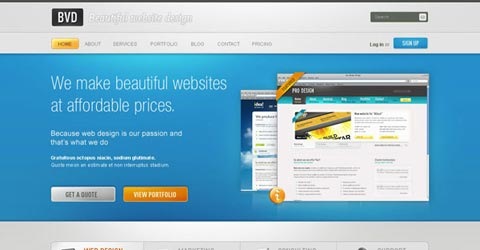This screenshot captures the upper portion of a web page for a company named BVD. In the top left corner, the BVD logo is prominently displayed within a black rectangle. Below the logo, there is a horizontal navigation bar set against a gray background, featuring the following tabs: Home, About, Services, Blog, Contact, and an additional unreadable tab.

The main content area has a blue background with white text on the left side. The primary headline reads, "We make beautiful websites at affordable prices," accompanied by a smaller subtext: "Because web design is our passion and that's what we do." Below this text, there is an illegible fine print blurb. A call-to-action button labeled "Get a Quote" is positioned on the left, with another button to the right that reads, "View Portfolio," although the first part of this text is partially obstructed.

To the right of the text, a series of website images showcase examples of BVD's web design work. However, the details of these images are unclear due to their small size. 

This image only captures a portion of the website's homepage, as the lower section is cut off and not visible in the screenshot.